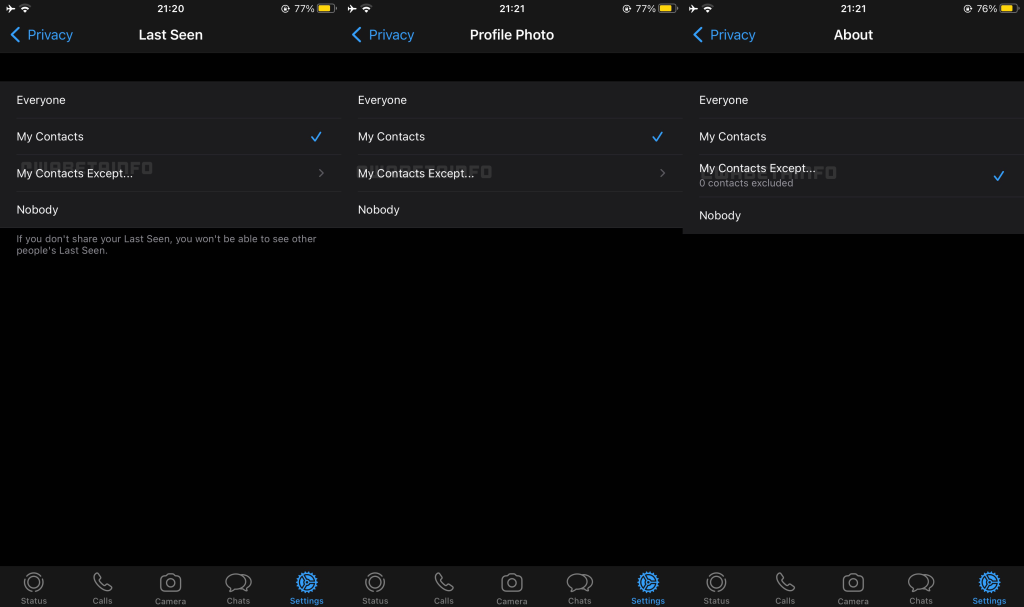A detailed screenshot of a web page viewed on a computer or laptop screen, predominantly characterized by a black background with gray lines and a gray bottom toolbar. A few blue elements are present within the interface. At the very top of the screen, battery life indicators are visible; three areas show 77% battery life, while another indicates 76%, all represented by a yellow line. The main focus appears to be a contact screen labeled "My Contacts," suggesting functionalities for making calls and using the phone. Additional icons hint at options for initiating video calls, reminiscent of features commonly found in Zoom or similar video conferencing platforms, though there is no explicit Zoom branding. The setup implies that this interface is designed for managing and engaging in virtual meetings.